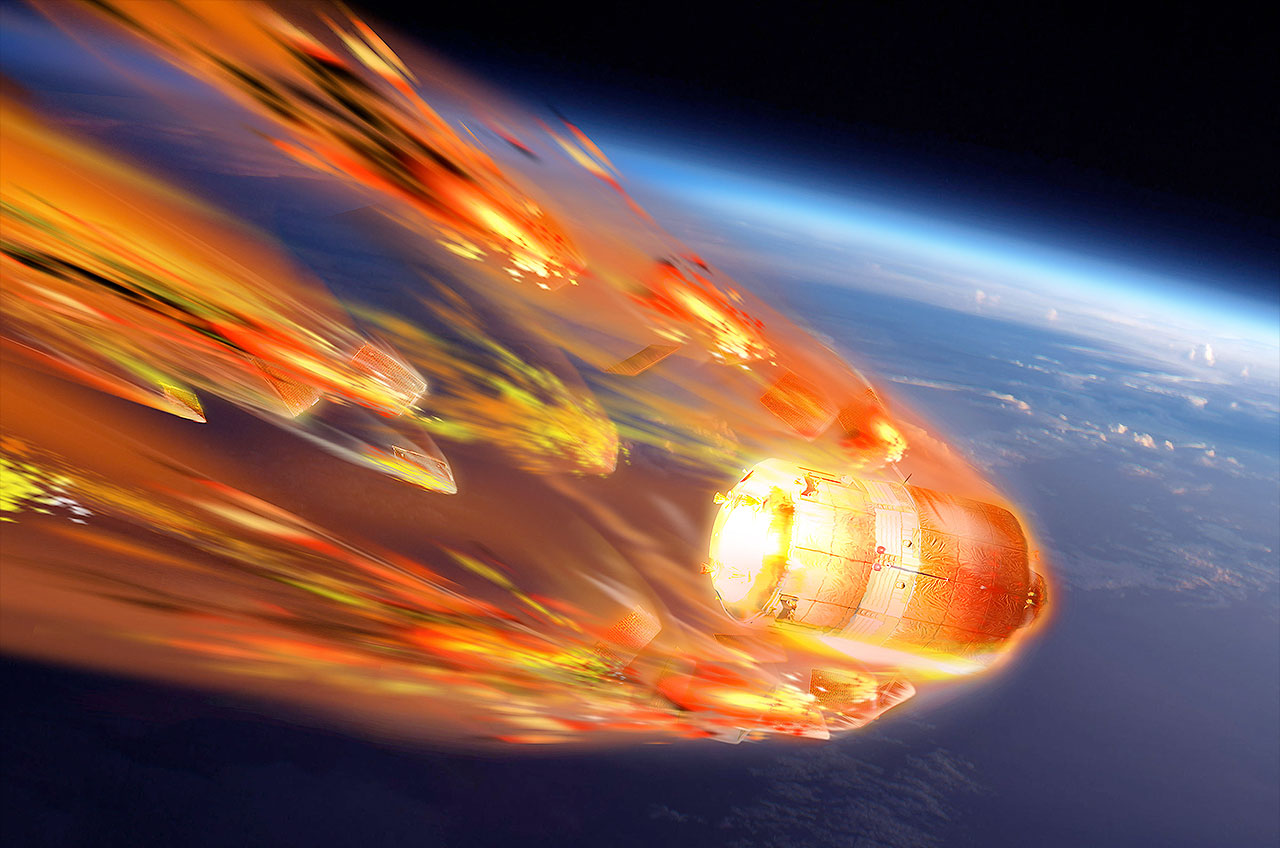A dramatic scene unfolds high above the earth, captured as if from the vantage point of an airplane. The focal point of the image is an oval-shaped cylindrical object barreling through the sky at what seems like incredible speed. The trailing end of this object erupts in an intense burst of orange and yellow flames, resembling an explosion. Below, the curvature of the Earth is visible, underscoring the significant altitude at which this photo was taken. This striking and dynamic image combines both the sense of rapid movement and high-altitude spectacle in a single breathtaking frame.